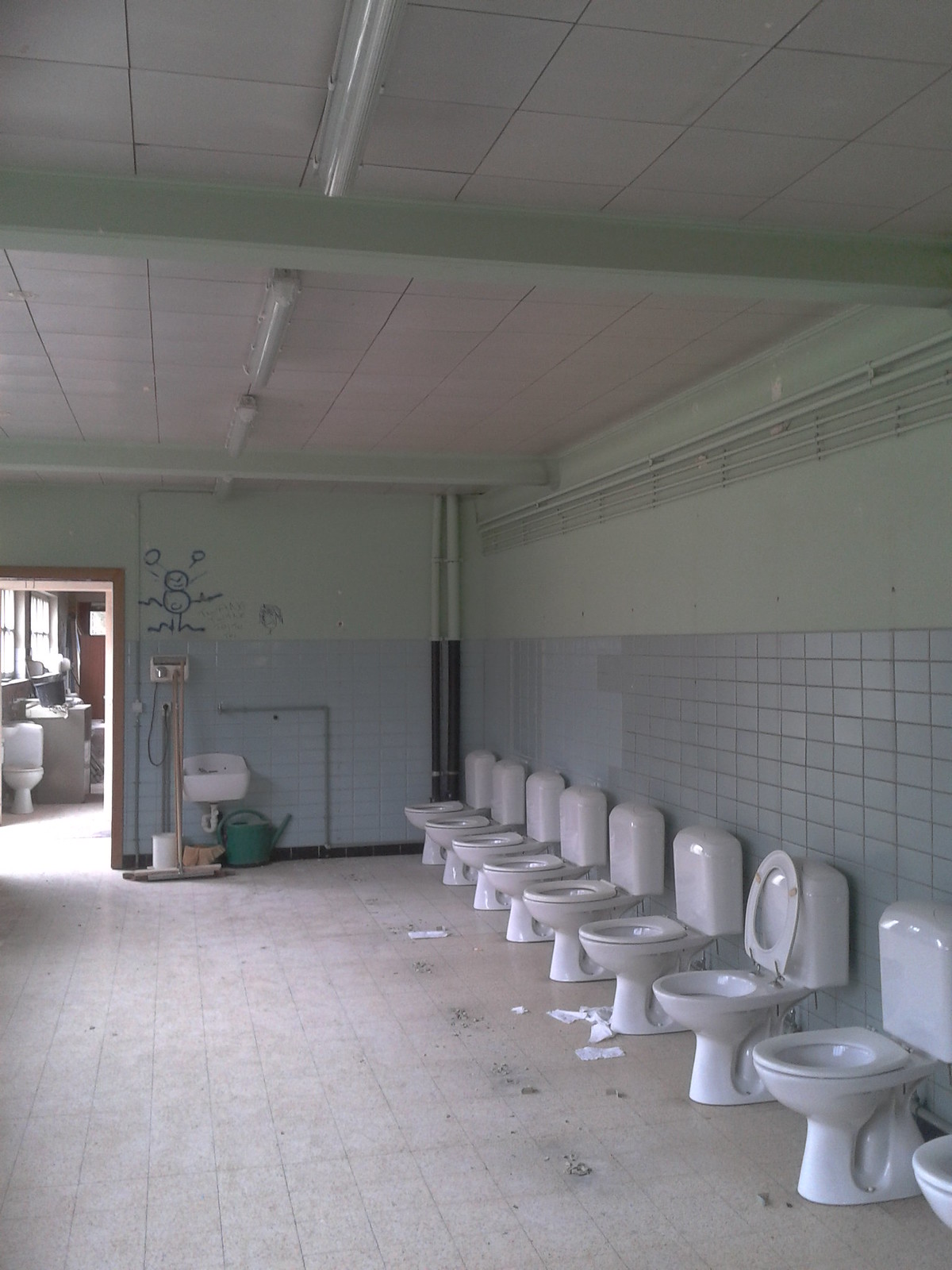This photograph provides a detailed view of a shared bathroom space, characterized by its unusual layout. The image captures the room from a vantage point close to one wall, facing a line of nine toilets arranged side-by-side with no dividers. The toilets, which have cisterns attached, are mounted against the right-hand wall of the picture. Notably, all toilet lids are closed except for the third one from the right.

The floor of the bathroom is covered in small, white square tiles, showing visible signs of discoloration from frequent use. Scattered around the fourth toilet from the right, there’s some toilet paper on the floor, adding to the slightly untidy appearance. The wall behind the toilets is tiled up to two-thirds of its height in rectangular, grayish tiles, transitioning to a pale mint green paint above.

The ceiling features a drop tile structure with large, white square tiles and three long, unlit tube lights running across it. Prominently, green beams support the ceiling, with one large beam extending from the right side nearly to the left corner, and another running horizontally at the far end of the room.

On the far wall, which is mostly lime green with a light blue lower half, there’s a hand dryer adorned with a blue drawing or graffiti above it. A door in the left corner is open, revealing another room with additional bathroom facilities and bright light streaming through. Two vertical pipes in the corner, colored light green at the top and dark green at the bottom, add to the industrial feel. Additionally, cleaning equipment and a sink are visible towards the back of the room.